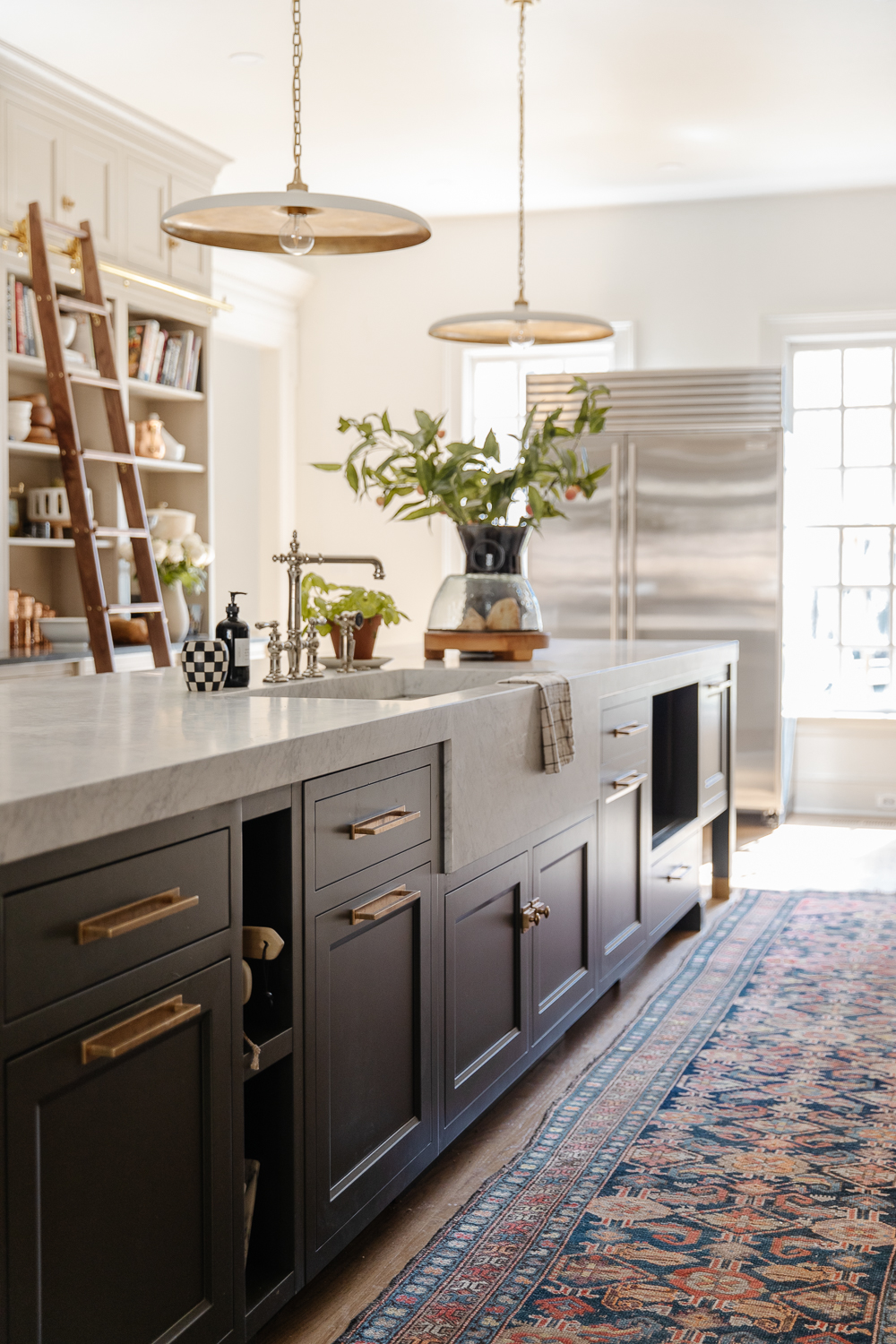This image depicts a spacious and modern kitchen with a predominantly white color scheme. Central to the scene is a large, white-topped island that houses a farmhouse-style sink. This sink, positioned in the middle of the island, has a dishtowel draped over its edge, and the sink area is adorned with several plants and a decorative checker print vase. The island features numerous dark brown drawers accented with bronze handles.

Flanking the stainless steel double-door refrigerator at the back are two windows, allowing natural light to filter into the room. Hanging above the island are two circular gold-colored pendant lights suspended by chains, illuminating the workspace below.

The floor is a light color, partially covered by a long, detailed rug running from the bottom right to nearly the middle of the right-hand side. The rug’s intricate design showcases a variety of shapes in vibrant blues, reds, and yellows. On the left side, there is an open pantry or bookshelf with multiple shelves filled with books and decorative items. A ladder is attached to this pantry for easy access to the upper shelves.

This image captures a blend of functionality and aesthetic appeal, characterized by the modern geometric design of the countertops and the ample storage space provided by the numerous cabinets and drawers.